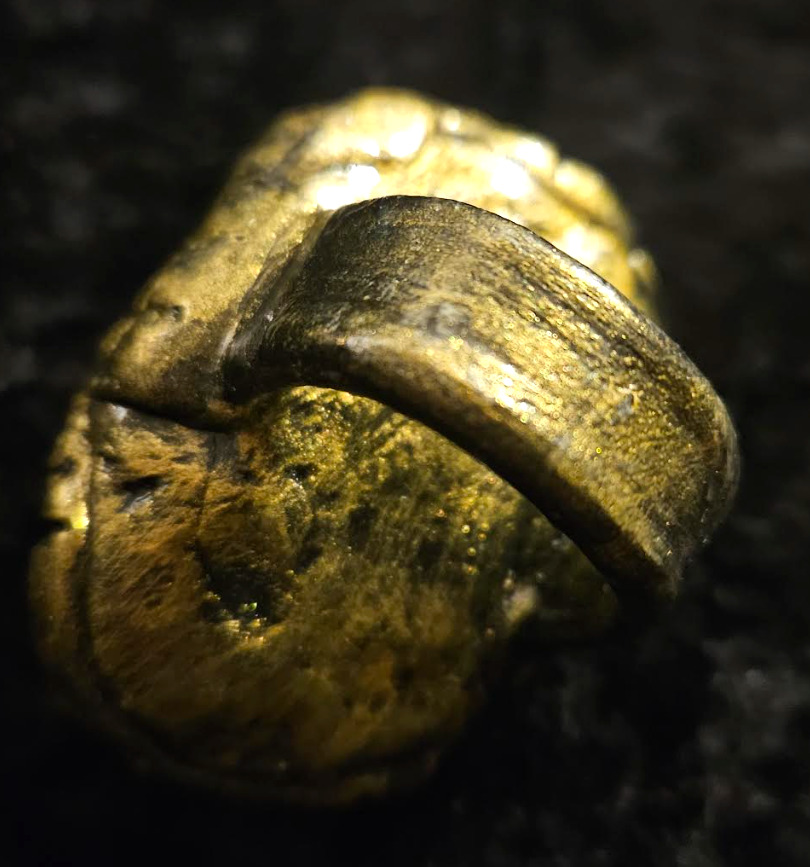This image features a highly zoomed-in close-up of a metallic gold object with a distinctly oval shape. The object is textured with a ridge that resembles a handle or handhold, and it has small black-speckled craters across its surface, giving it a rugged appearance. The golden color varies in intensity, appearing more yellowish and shiny where the light hits it and darker in the shadows. The highly reflective and glittery background is a mix of dark black and grays, making the object stand out prominently. Due to the extreme close-up, the actual size and true nature of the object remain ambiguous; possibilities range from a piece of metal or brass to potentially a piece of jewelry like an ornate, thick-banded ring.